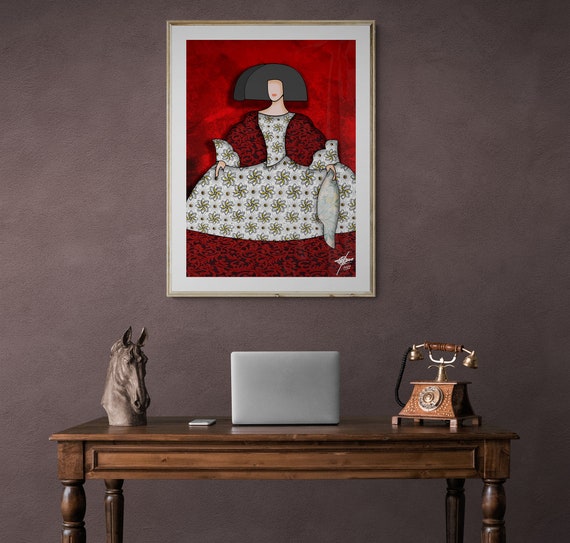This image captures a foyer or entryway featuring a dark wood table with four legs against a dark-toned wall, which could be very dark blue, green, or black. On the table, in the center, is a mysterious gray or silver cube-like object. To the left is a detailed sculpture of a horse's head, predominantly gray, showcasing just the snout and pointy ears. To the right of the cube sits an old-fashioned telephone, characterized by its orange and gold, or perhaps copper, finish, designed to resemble vintage telephones with a cradle. 

On the wall behind the table hangs an intricate painting of a woman. She has shoulder-length, voluminous black hair and is dressed in a very puffy and elaborately patterned gown. Her dress features colors like white, blue, and yellow, adorned with starry or snowflake-like patterns. She also wears a dark red shawl over her shoulders. The painting's background is a bold red with a distinctive white border, making the artwork stand out vividly against the dark background of the wall. This detailed setting combines classic and contemporary elements, creating a striking yet cozy atmosphere.